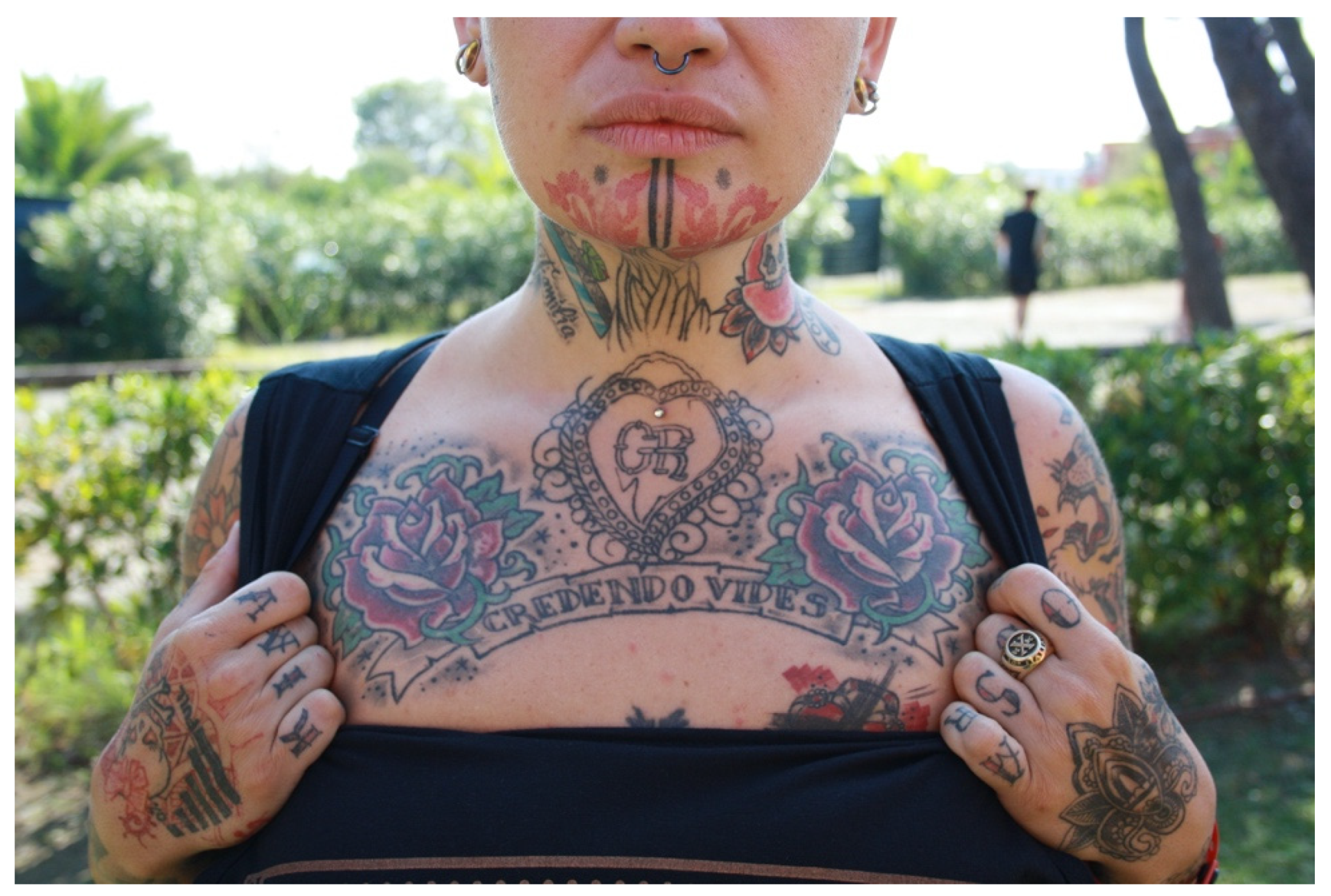The image is a detailed, well-lit photograph taken outdoors during a sunny day, featuring lush green vegetation such as grass, bushes, and trees. The primary focus is on an individual, likely a woman, showcasing her tattoos. The image captures her from about the upper chest to just below her nose, excluding her eyes. She is dressed in a black, strapped top and is using her hands to pull the straps apart, revealing an intricate tattoo on her upper chest. This tattoo features a heart with the initials "GR" in the middle, flanked by red roses and green leaves. Below the heart and roses, a ribbon stretches across her chest with the phrase "credendo vides" inscribed on it. Additional tattoos are visible on her chin, neck, shoulders, and the backs of her hands, which also display tattoos with the letters "AV" (or "KIAV") and "AAS." She has gauged earrings and a septum piercing. In the background, a blurred figure of a man can be seen amidst the verdant surroundings.